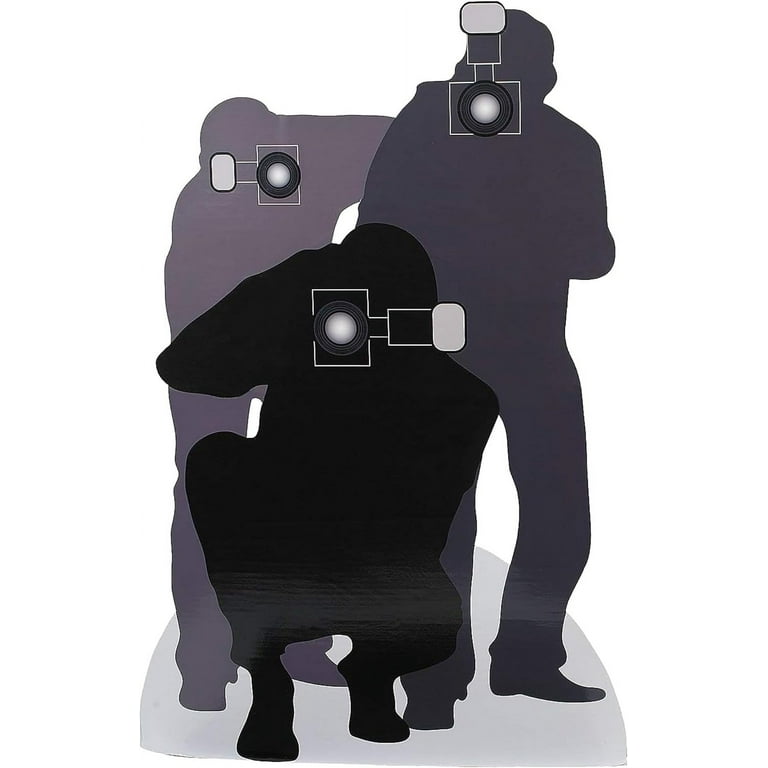The image features the silhouettes of three men in various poses, resembling cutouts of paparazzi. The figures are in different shades of gray: the leftmost is light gray, the middle one is a darker gray, and the rightmost is almost black. All three silhouettes hold camera-like devices in front of their faces, aiming them towards the viewer. The man on the left stretches his left shoulder or arm outward, partly obscured by the middle figure who stands in a slightly hunched position. The third figure, positioned in front, is crouching with what appears to be bare feet. Notably, the scene includes a gray semicircle on the ground near their feet, enhancing the effect of the silhouettes. The lack of facial features, clothing details, and explicit camera flashes emphasizes their shadowy, almost ghostly presence as they capture the moment.